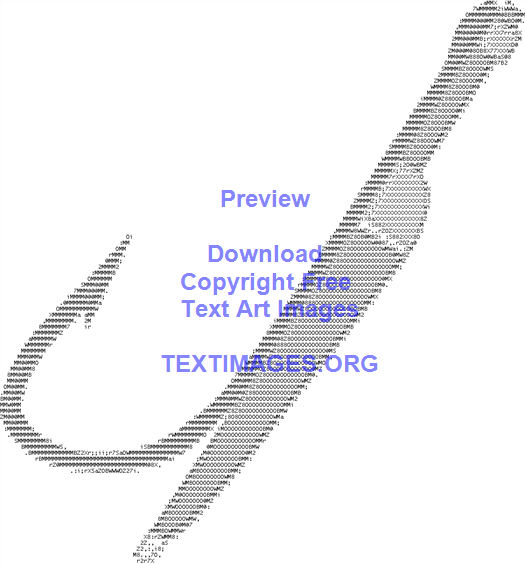This is a scan of an intricate piece of text art that depicts a fishing hook attached to what appears to be either a knife or a pen. The fishing hook is illustrated pointing upward, while the pen or knife is shown beneath it. The artwork is crafted entirely from strategically placed letters and numbers, creating varied shades of black and gray, with some areas appearing darker due to bolder typeface. The detailed design is set against a stark white backdrop. Centrally overlaid in blue text, the words "preview download copyright free text art images textart or textimages.org" are prominently displayed. The only distinct color in the image is the blue text, which serves to guide viewers to the source of the text art. This ASCII art, viewed as if it forms a cohesive tool, masterfully combines both graphical and text elements, with the letters and numbers densely packed in certain areas to create a tangible depth and dimensionality.